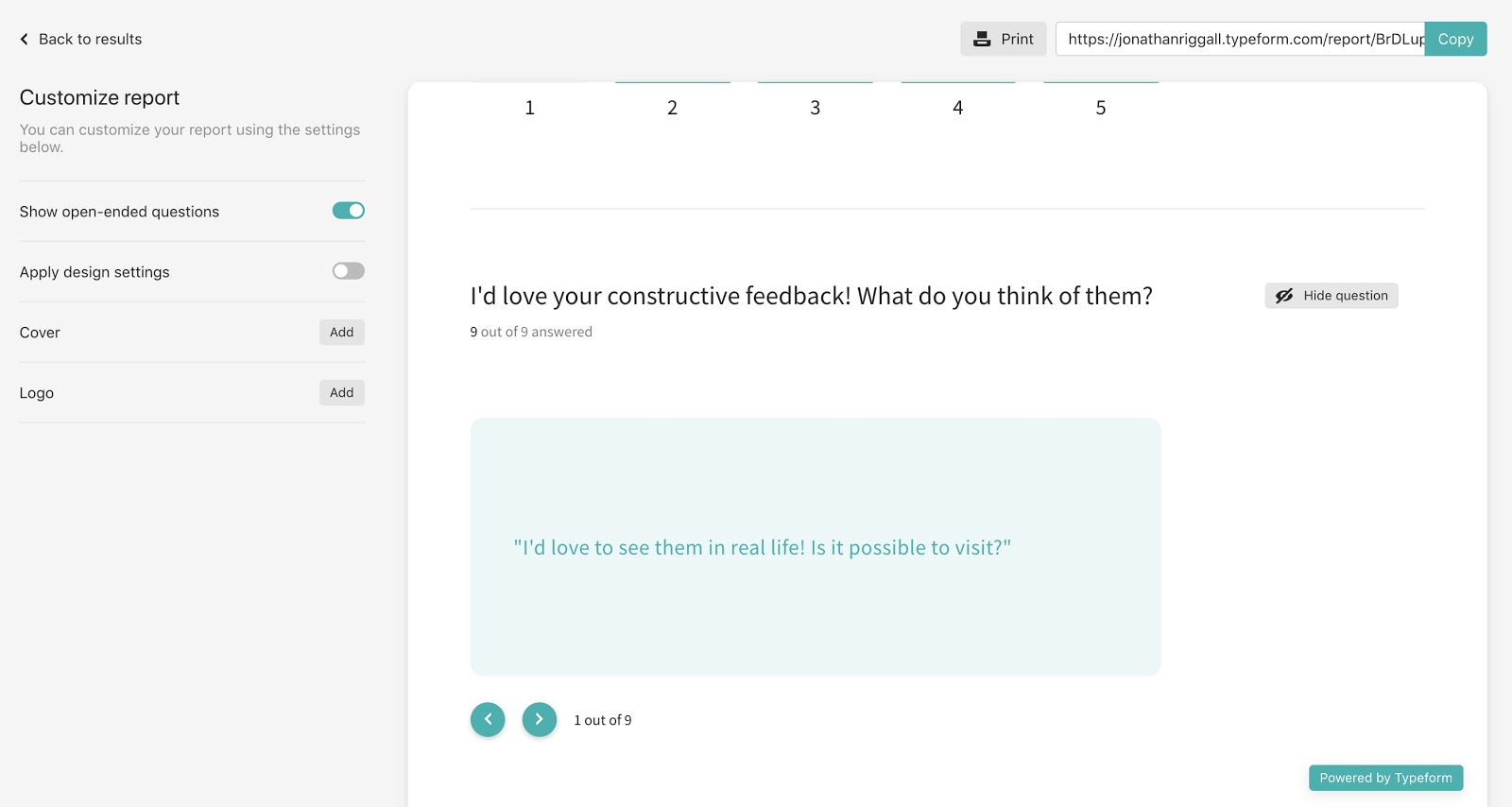An image displays two screenshots of a survey report interface from a Typeform page. The upper screenshot features a gray background with a navigational bar at the top containing options: "Back to results," "Print," the site name, and a green "Copy" button. On the left, the text "Customize Report" is shown, followed by instructions saying, "You can customize your report using the settings below." Several toggle options are listed: "Show open-ended questions" (enabled), "Apply design settings" (disabled), "Cover" (disabled), and "Logo" (disabled).

The lower screenshot is set against an all-white background. At the top, numerical labels from one to five are laid out in written form. Beneath this, the text reads, "I'd love your constructive feedback. What do you think of them?" with a notation indicating "Nine out of nine answered." Directly below, a response box shows a single piece of feedback marked by "I question," with one out of nine results highlighted in a green box containing the response, "I'd love to see them in real life. Is it possible to visit?" To navigate through additional responses, there are green arrow buttons on either side to cycle left or right. At the bottom right corner, there is a "Powered by Typeform" stamp, indicating the source of the survey interface.